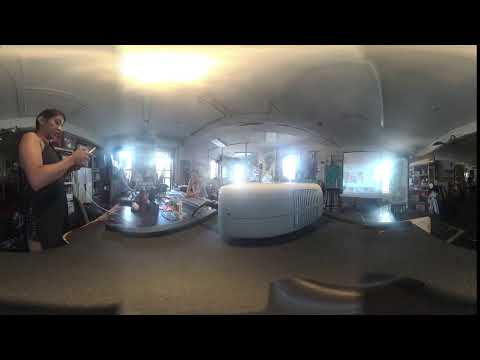The image is a horizontally aligned, rectangular photograph with thick black borders on the top and bottom. The picture is somewhat blurry, capturing a bright daylight scene through several windows in the background. Standing towards the back is a man in a blue top and dark pants, though his details are indistinct due to the blur. In the foreground on the far left, a woman is seen from her right side. She has brown hair pulled back and is wearing a sleeveless black top along with dark bottoms, possibly a tank top or a dress. She's intently looking down at an object in her hands, which could be a pen, notepad, phone, or tablet.

The scene appears to be set in a bar or workshop with a counter in the center. On the counter sits a white device with vents at the back and a cord running out of it, possibly an air humidifier or another small appliance. The counter itself is black and may have stools against it, suggesting it is a bar top. Despite the bright light shining through the windows and obscuring some details, the ceiling is clearly white, and additional people can be faintly seen sitting further down the counter, adding to the bar-like atmosphere. The woman might be bartending, focusing on her task amidst the blurry, softly lit surroundings.